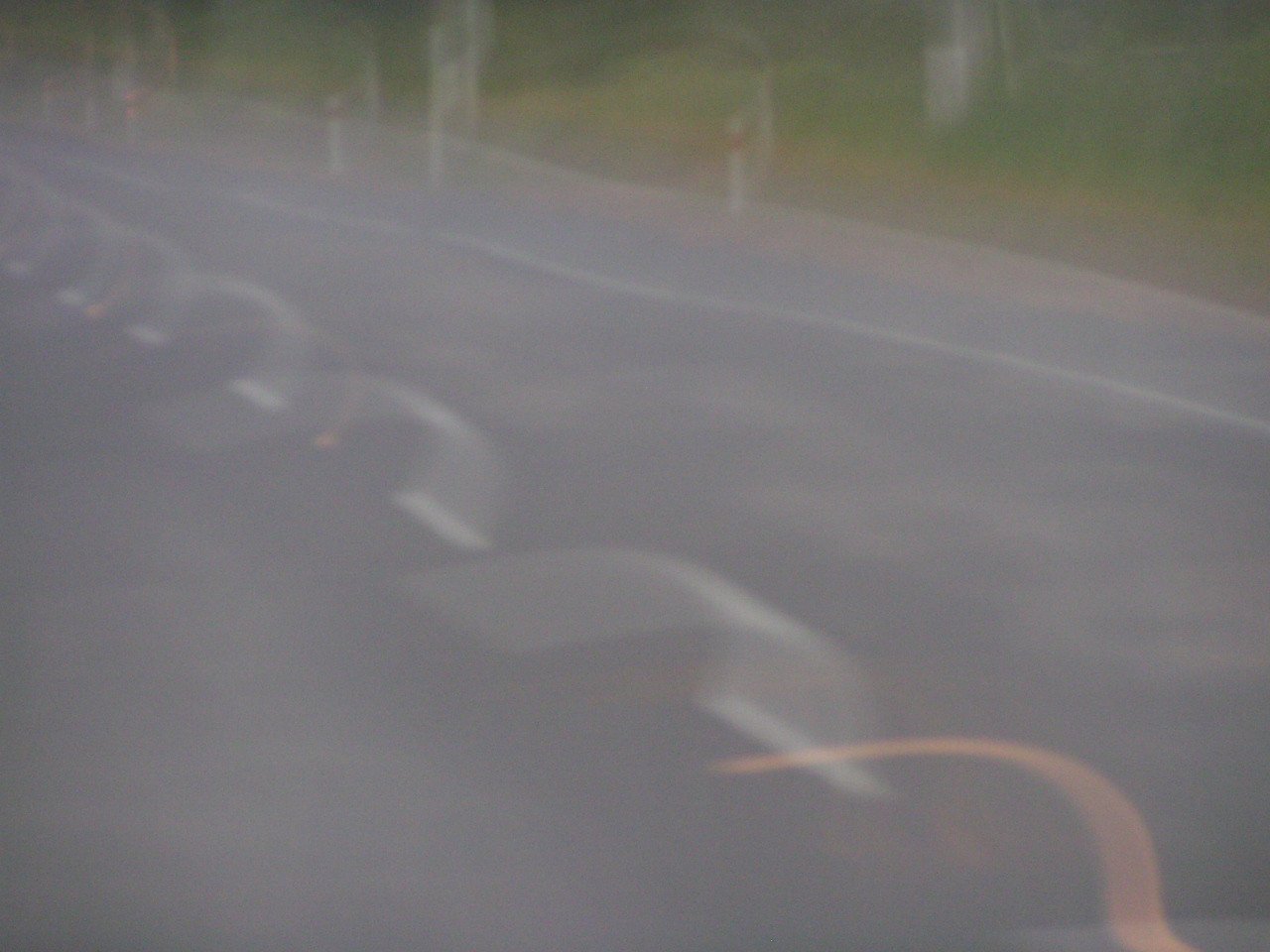The image depicts a very blurry, distorted view of a two-lane asphalt road. The motion blur suggests the photo was taken at high speed or with some camera movement, resulting in an interesting pattern where the normally straight, dashed white lines in the middle of the road appear as curved, arch-like trails. The solid white line on the right side of the road also follows this distorted effect. The road, viewed at a 45-degree angle, shows a lack of cars, adding to a sense of quietness. The surrounding area includes a green bank or the start of a hill on the top right, along with some gravel and grassy patches. There's an indistinct orange blur at the bottom right of the image, adding to the chaotic motion effect, and a hint of gray pillars that could be traffic or power line posts along the right side of the road.